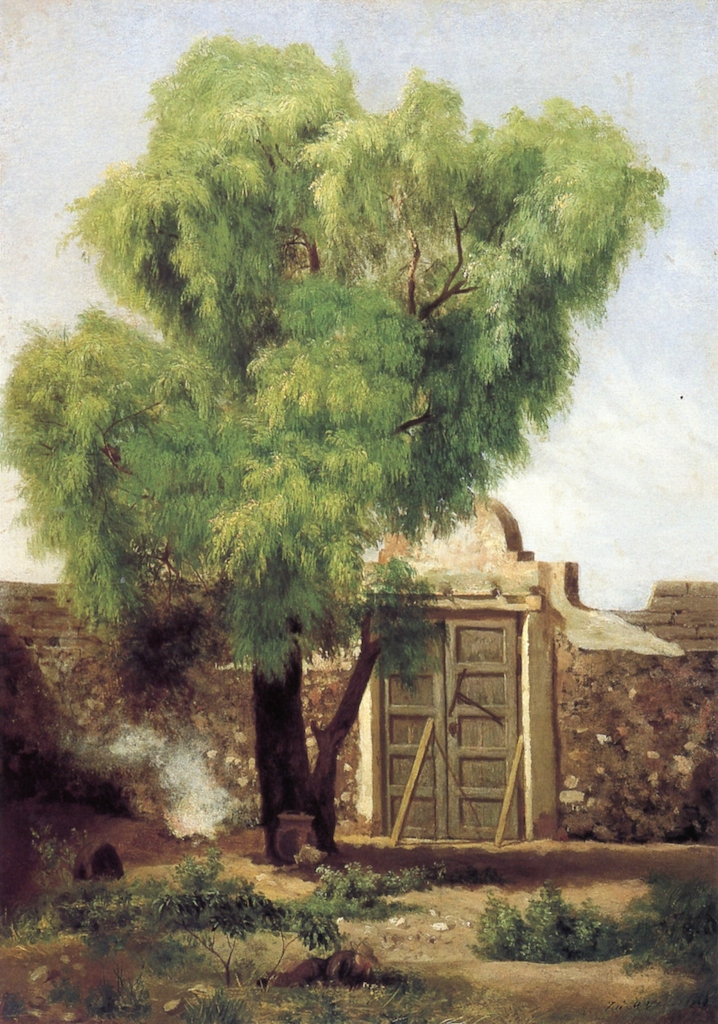The painting captures a serene, bucolic outdoor scene under clear blue skies. Central to the composition is a tall, lush green tree casting a substantial shadow, indicative of the bright sunlight. At the foreground, a person in a brown suit lies on the grass wearing a straw hat, seemingly resting or leisurely observing the surroundings. There are areas of light dirt and shrubbery interspersed on the ground. Under the tree, partially enveloped in shadow, is a large pot adding to the rustic charm of the setting. Behind the tree stands a sturdy gray brick wall with a closed wooden gate, propped shut by two wooden planks. The wall features a decorative cement top that rises above the gate. The vibrant summer foliage and the detailed depiction of light and shadow suggest a hot and bright day.